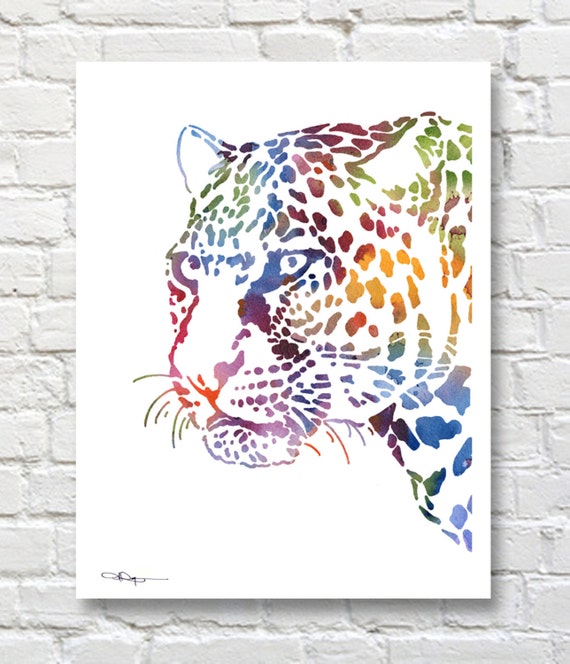The photograph, vertically oriented and shot indoors, showcases a striking piece of artwork mounted on a white brick wall. The central subject of the canvas is a vividly colored depiction of a tiger's face. The artistic representation features intricate details with diverse colors such as orange, green, blue, purple, red, and gray, creating a unique, speckled effect instead of traditional fur. The tiger, or possibly a leopard, is characterized by small ears, expressive eyes, a prominent nose, and a detailed mouth. The white background of the canvas highlights the colorful animal, making it stand out. Positioned on the lower left side of the canvas is the artist's signature, adding an authentic touch to the vivid drawing. The white brick wall background, with its clear outlines, complements the overall aesthetic of the artwork, centralizing and emphasizing the detailed and colorful nature of the piece.